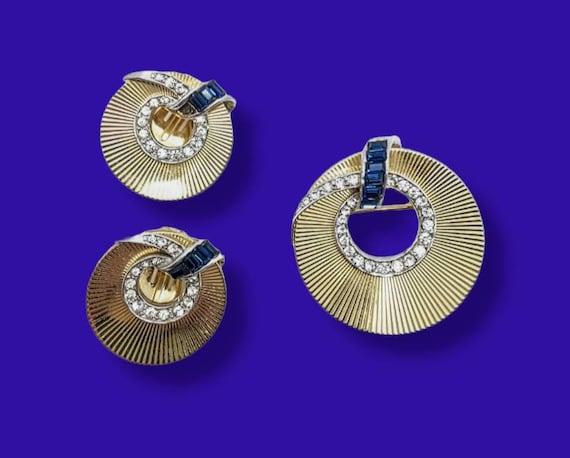The rectangular image features a rich navy or royal blue background that is wider than it is tall. Positioned on this bold backdrop are three intricately designed jewelry pieces that resemble pins or pendants, which could potentially adorn an article of clothing. These pieces are circular and crafted from gold, with two smaller ones on the left and a slightly larger one on the right. The distinct detail shared by all three is their swirling, staircase-like design that incorporates a line of diamonds encircling the center. Each piece also features strikingly blue gemstones arranged in a segment at the top, which add a vivid contrast to the golden hue. The top left and right jewelry pieces are of a lighter gold color, while the one on the bottom left is of a darker golden shade. The array of blue stones, potentially sapphires, complements the central diamonds, enhancing the intricate beauty of these three artifacts displayed against their vibrant blue setting.